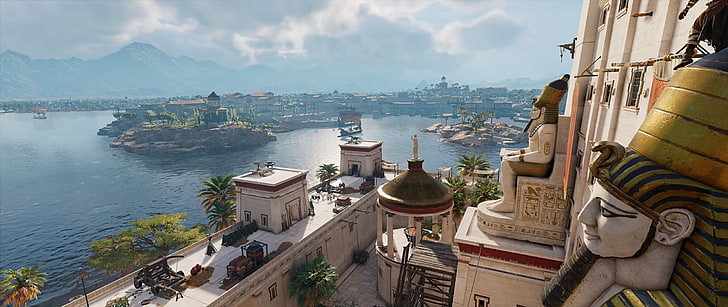This stunning photograph captures the majestic exterior of an ancient Egyptian tomb. Dominating the foreground, two grand statues of pharaohs are seated in front of the entrance, each meticulously carved from stone and adorned with vivid gold and blue paint. The pharaohs sport elaborately painted black beards, adding to their regal appearance. 

Beyond the tomb, the photograph opens up to reveal a breathtaking panorama of the surrounding area. A shimmering, bright blue body of water contrasts strikingly with the arid landscape. Nestled closer to the water, a smaller building or temple can be seen, its presence overshadowed by the grandeur of the sprawling cityscape in the background. 

The city is a maze of buildings, houses, and various structures that stretch far into the horizon. Rich greenery embellishes the scene, with lush trees and iconic palm trees standing tall. In the background, a range of dark blue mountains forms a natural boundary, adding depth and a sense of scale to the composition.

The sky overhead is almost entirely clear, painted in a vibrant shade of blue. However, on the left side, wispy, medium-gray clouds float by, breaking the uniformity of the sky and adding a touch of texture to the image. Overall, the photograph beautifully captures the magnificence and historical richness of the ancient Egyptian landscape.